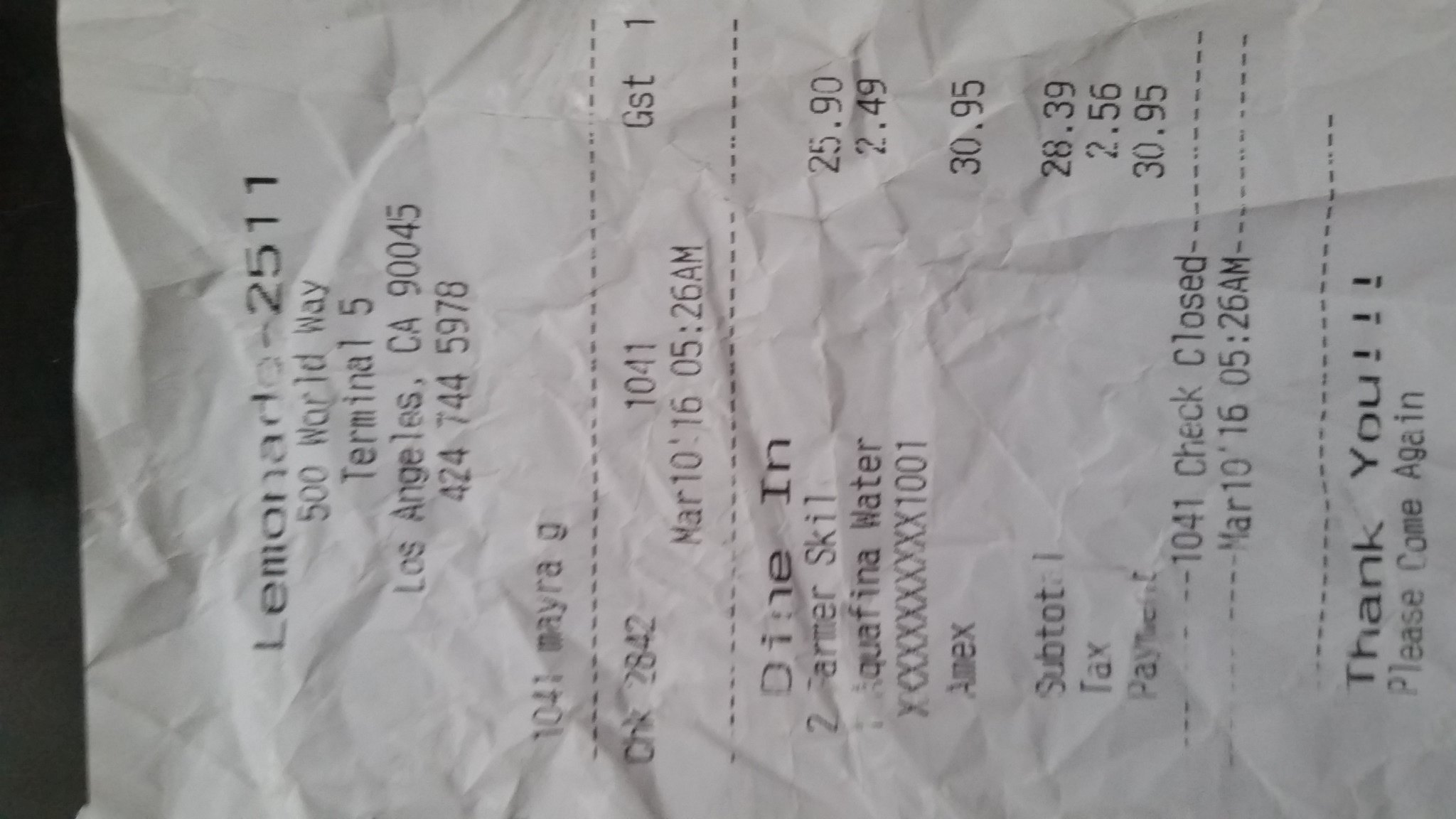This black-and-white photograph offers an intriguing close-up view of an old-fashioned register receipt, printed on traditional register paper. The receipt is oriented sideways in the image, requiring viewers to tilt their heads to read its details. At the very top, the receipt prominently displays the establishment name: "Lemonade 2511." Beneath this, the address "500 World Way, Terminal 5, Los Angeles, California" is clearly printed, followed by a contact phone number: "424-744-5978."

The date of the purchase is listed as March 10th, 2016, at precisely 5:26 a.m. Indicating that the patrons dined in, the receipt further specifies that the meal took place at the lemonade venue within an airport terminal. The transaction culminates in a total amount of $30.95, reflecting the cost of the meal enjoyed on that early March morning.